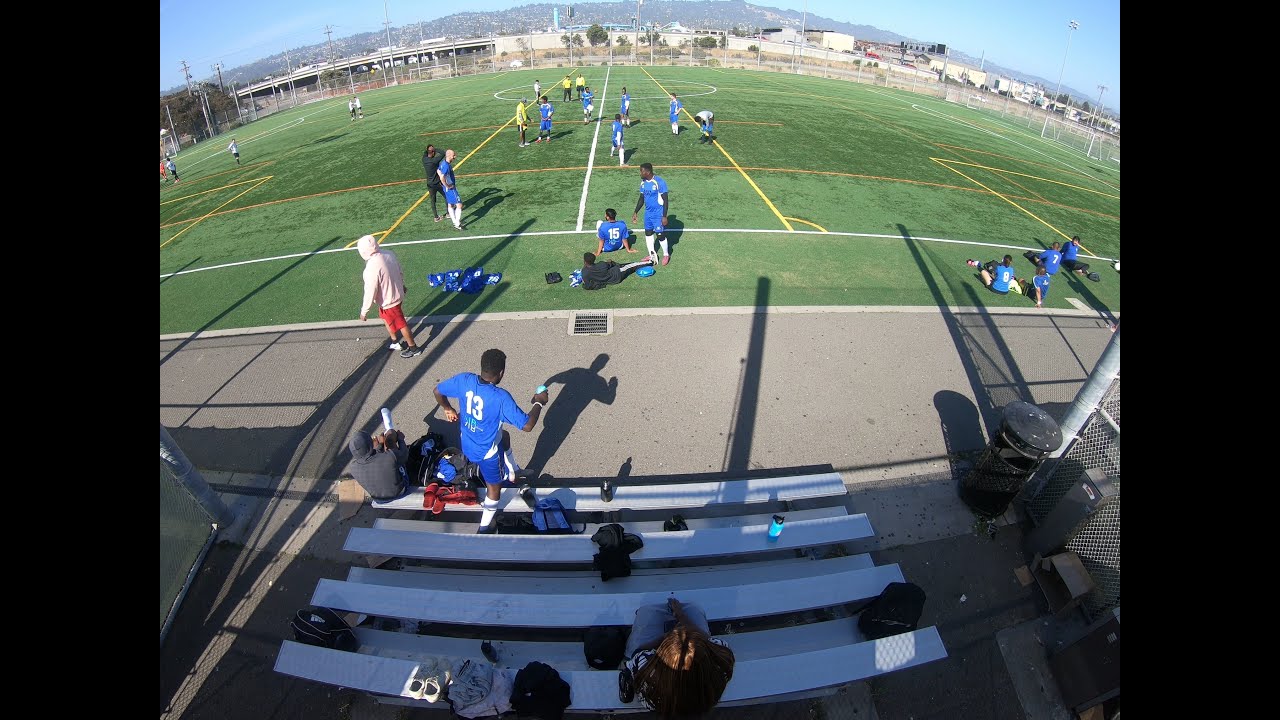The image captures a vivid and dynamic scene at a sports field, presumably during a soccer game or practice. The photo is taken from a high vantage point, possibly a GoPro with a fisheye lens, which gives the scene a panoramic feel. In the foreground, white bleachers are visible, with several people sitting on them and backpacks scattered around. A man in a blue jersey with the number 13 on the back is descending the white stairs adjacent to the bleachers.

The large, green field features a white line near the boundary, yellow lines toward the center, and a distinct white circle in the middle. Numerous players are on the field, predominantly dressed in blue jerseys and shorts. Three players wear yellow tops and black pants, adding some contrast. A person in a pink hoodie and red shorts stands out among the spectators. 

In the background, past a fence enclosing the field, lies a cluster of buildings with a towering mountain range behind them. The sky above is clear and blue, dotted with a few white clouds, while the sun shines brightly, illuminating the entire scene. The detailed backdrop includes houses nestled on the mountains, a bridge, and several power lines, contributing to the vibrant and bustling atmosphere of the image.